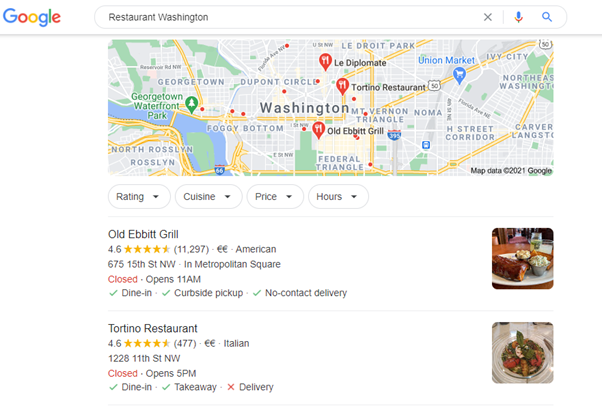The image being described appears to be a detailed screenshot or mockup of a restaurant search result page on Google Maps. Here is a cleaned-up and detailed caption for the image:

---

The top left corner of the image displays the Google logo. The top part of the interface features various icons including "Restaurant" on the left, followed by an "X" icon, a microphone icon, a magnifying glass icon, and a map icon that indicates the location is Washington, D.C. Within the map section, key locations are marked, such as Georgetown Waterfront Park, Georgetown, Dupont Circle, and pins indicating locations like Lid DuPont, Tortina Restaurant, and Old Epic Grill.

To the right side, there's a list that includes H3 Corridor, Carver Links, Northeast Washington, Ivy City, Margalla Drive Park, and more, in addition to neighborhoods like North Rosslyn, Rosslyn, and Federal Triangle. 

Further details about two specific restaurants are provided. The first is "Old Epic Grill," which holds a rating of 4.6 stars from 11,297 reviews. It serves Euro-American cuisine, with specific mentions of Durian and Chesapeake cuisine, and side dishes. Located at 675 15th Street, Northwest, in Metropolitan Square, it opens at 11 am and offers dining and no-contact delivery services. 

The second restaurant, "Tortina Restaurant," also has a 4.6-star rating from 477 reviews and specializes in Italian cuisine. It is situated at 1, 228 11th Street, Northwest, and opens at 5 pm, offering dining but no delivery service. The background color of the interface is predominantly white.

---

This refined caption provides a detailed and structured description of the image, including key details about the restaurants and their location context.